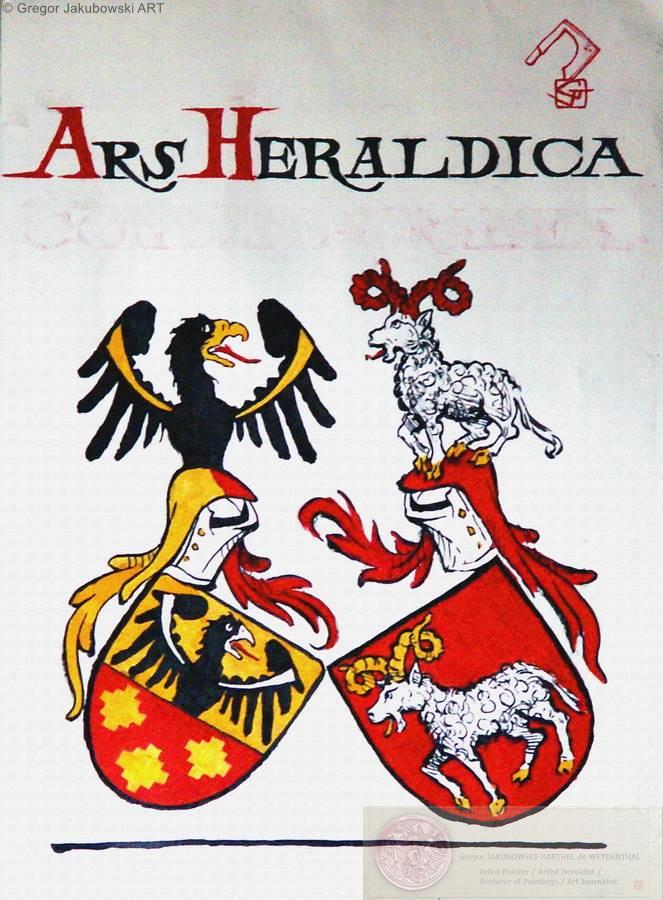The image depicts a detailed coat of arms featuring two crests. The left crest showcases a black bird with white stripes on the bottom of its wings, its beak open, and its tongue protruding, against a yellow background. Beneath the bird, three diamond-like shapes are placed on a red background. The right crest displays a white ram or sheep with large yellow horns and yellow hooves, set against a red background. Above these crests, the same black bird and white ram are mirrored, symbolizing their importance. The crest is topped with the text "Ars Herotica," with the 'A' in 'Ars' and 'H' in 'Herotica' highlighted in red. In the top left corner, the text "Gregor Jakubowski Art" is visible along with a copyright symbol. Additionally, a circular red watermark is located at the bottom right, and a small, red sickle-like drawing is present at the top right. The colors black, white, red, and yellow dominate the composition, enhancing its heraldic presence.